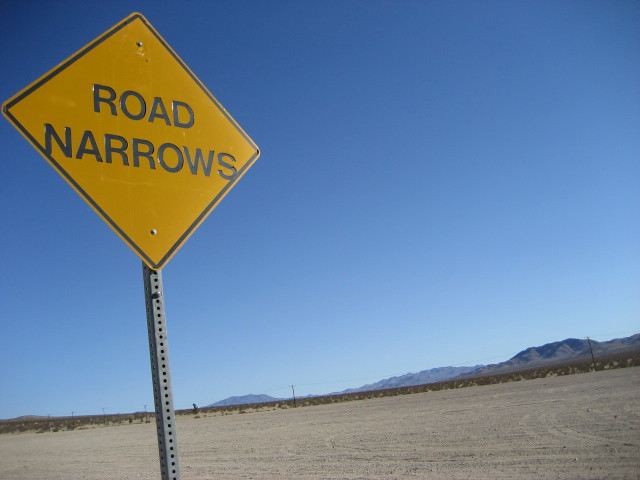This image captures a stark desert landscape under a bright, expansive sky. In the foreground, a solitary steel pole supports a yellow diamond-shaped road sign with the black-lettered warning "Road Narrows." The ground beneath the sign is flat, unpaved, and covered in sparse desert vegetation, characteristic of the arid environment. Behind the sign, the vastness of the desert stretches out, showing a gradual transition from brown dirt to sparse greenery further back. A small fence peeks out in the middle distance, while electrical poles and lines punctuate the scene, adding a touch of human presence. Far in the background, a rugged mountain range undulates across the horizon, its peaks and valleys silhouetted against the sky. The sky above is a gradient of blues, transitioning from a lighter tint near the mountains to a deeper hue as it rises, suggesting a clear and sunny day.